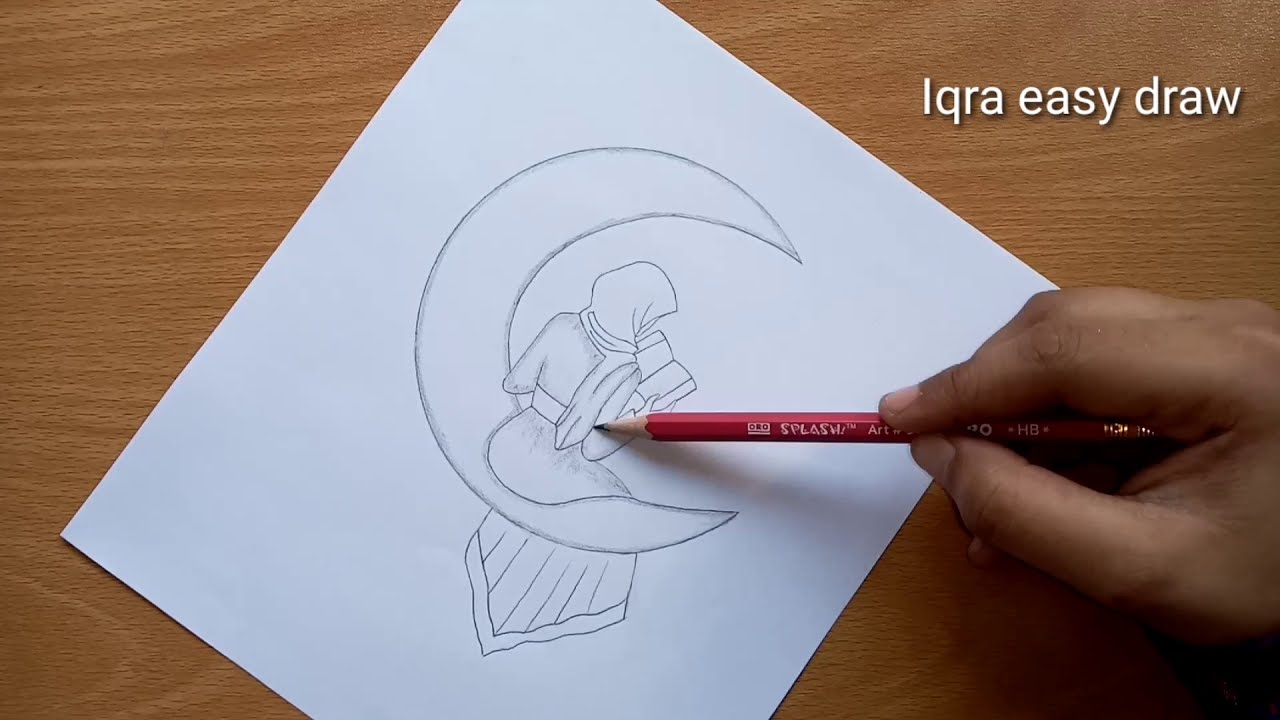The image appears to be a screenshot from a video tutorial on how to draw. Set against a medium-toned wooden table backdrop with visible wood grain running left to right, there is a white piece of paper laid out in the center. On the paper is a pencil sketch depicting a crescent moon, lightly shadowed, with a woman sitting on it. She is wearing traditional Middle Eastern attire, including a hijab, and her dress flows elegantly over the moon's edge. The woman has a sash around her waist and is engrossed in reading an open book. A man’s hand, with brown skin, is visible on the right side of the image, holding a sharpened red pencil against the paper, seemingly pointing at the sketch. In the upper right corner of the image, text reads "IQRA Easy Draw," suggesting that this is an instructional guide for drawing the depicted scene.